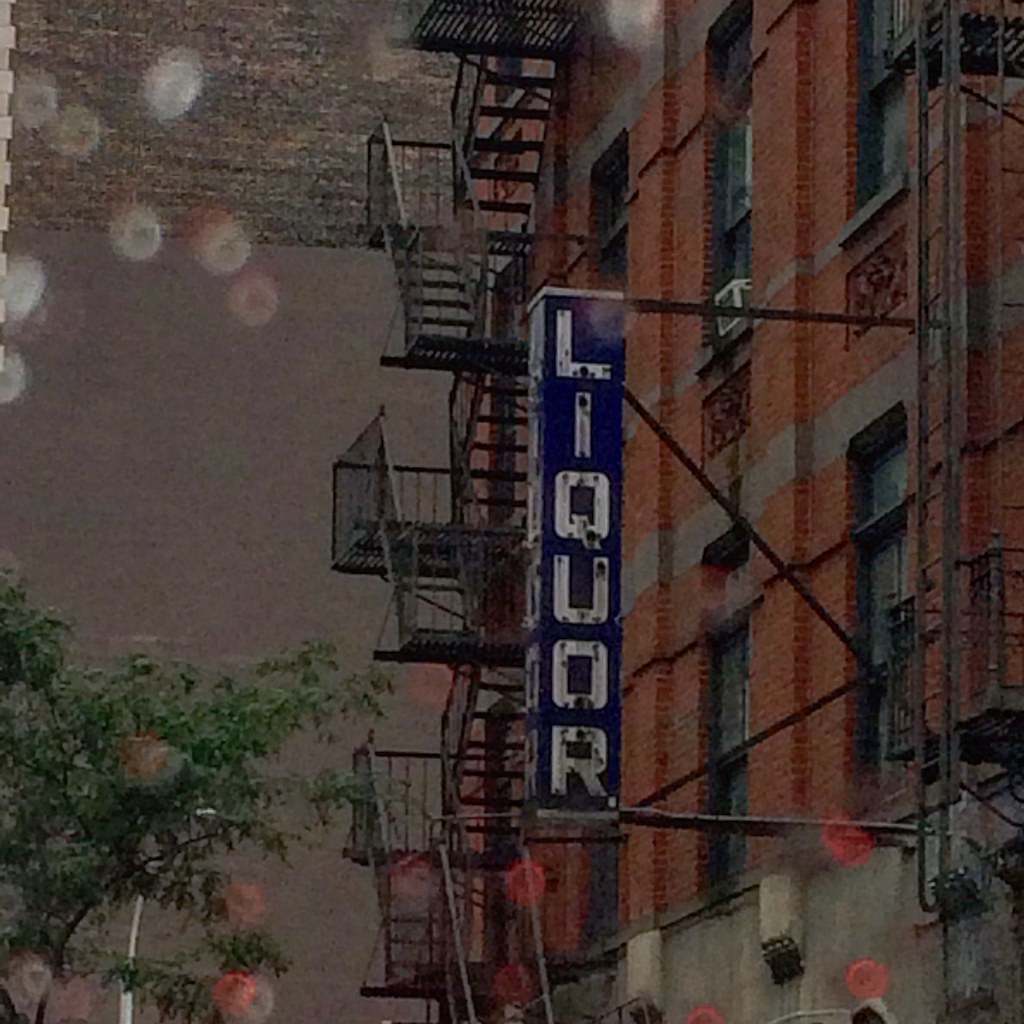The image depicts an older red brick apartment building, distinguished by its extensive fire escapes that zigzag from the ground to the roof. It stands adjacent to a gray brick building and is likely set in an urban environment. The scene, captured either through a hazy photograph or a painting, is accentuated by a rainy ambiance, evidenced by splatters of rain on the lens and dark gray skies. A prominent, weathered sign reading "LIQUOR" in white letters on a blue background is affixed to the red brick building, extending vertically from steel brackets. In addition to the fire escapes, a single large steel ladder is attached to the building. A tree and a large lamppost can be seen on the left side, adding to the cityscape's character. The lower portion of the building features cement-colored sections, while sporadic lighting reflections create white and pink spots, adding a dynamic, almost mystical quality to the overall composition.